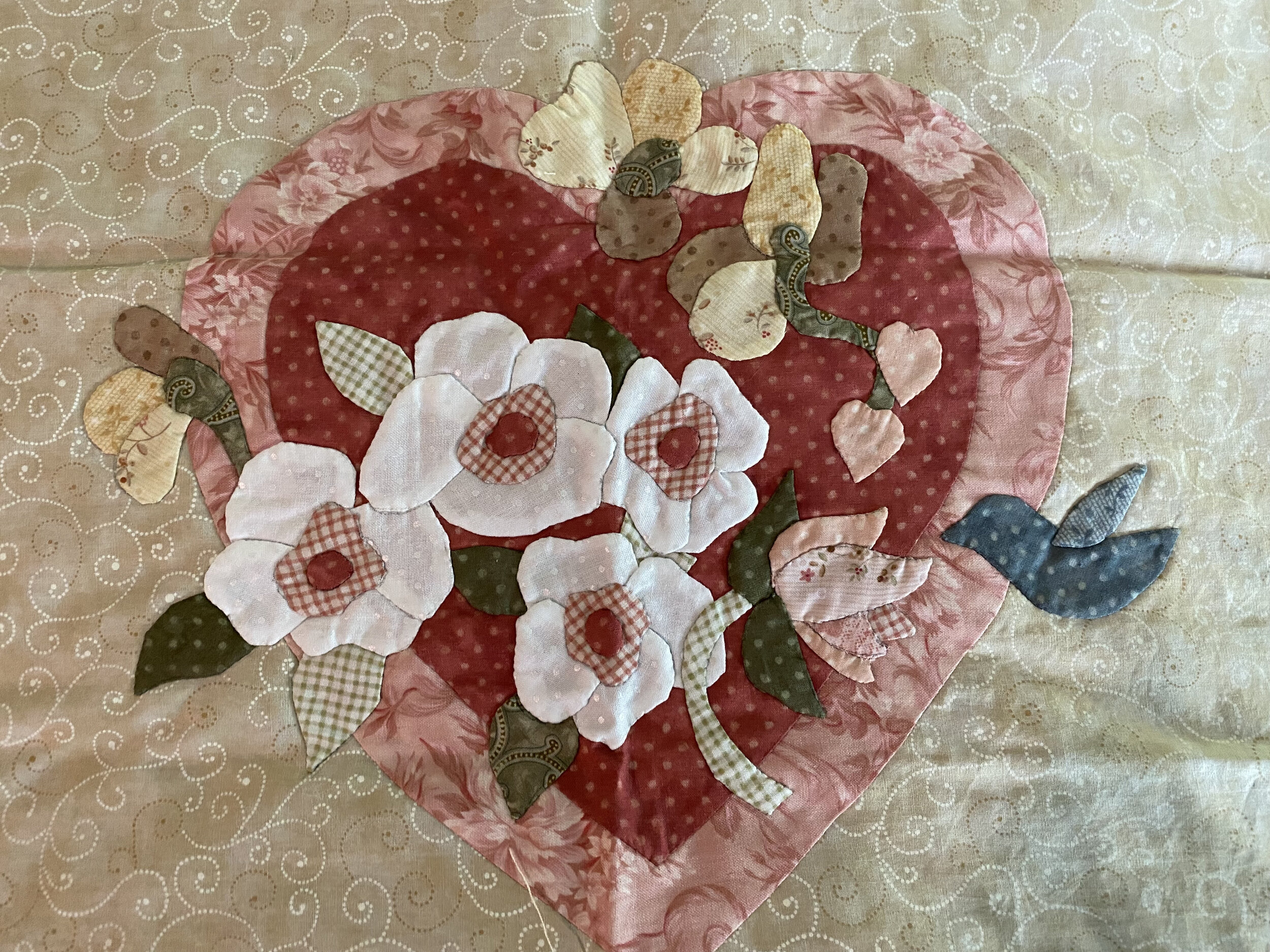The photograph captures a detailed, handcrafted quilt featuring an intricate applique design. The quilt is cream-colored with a subtle white scroll print pattern as its base. At its center, a large heart applique stands out, meticulously sewn from different fabrics. The heart is made from dark red fabric adorned with white dots, and it is framed by a border of pink fabric with beige rose prints. Inside the heart, a variety of flowers are arranged: a cluster of white flowers with red and white checked centers and red buttons, cream-colored flowers with beige accents, and smaller pink hearts. A gingham-checked stem supports one of the blossoms. 

To the right of the heart, a small blue bird appliqued from dark blue fabric with light blue wings perches, facing the heart. This bird adds a charming touch to the scene. The applique extends beyond the heart's borders, integrating the design seamlessly into the quilt. The quilt also shows visible crease lines from folding, emphasizing its tangible, handmade nature. The photograph, taken in landscape orientation, highlights the meticulous craftsmanship and the harmonious blend of colors and patterns, presenting a piece of photographic representationalism realism.